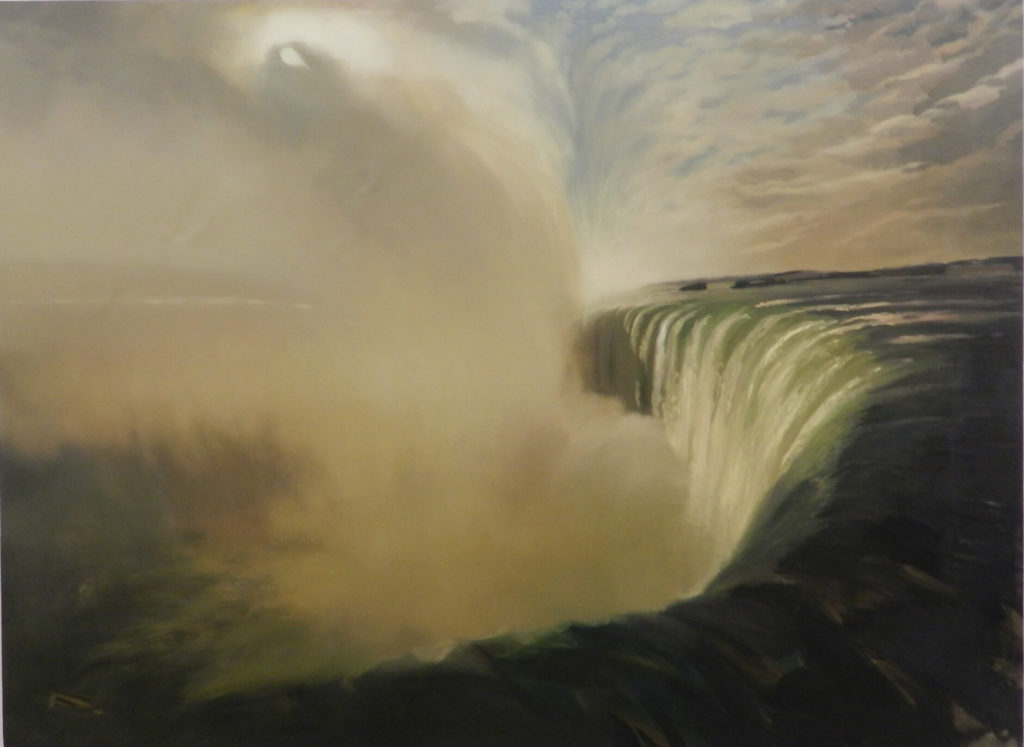The painting depicts a vast, majestic waterfall cascading off a steep cliff, dominating the lower two-thirds of the square canvas. The massive volume of water pours over the edge, creating a powerful sense of being right at the precipice. A swirling mist rises up from the waterfall, forming dense, round clouds that ascend and mix with the feathery clouds above, almost mimicking a genie emerging from a bottle. The upper third of the image features a sky dotted with patches of blue and an array of white and gray clouds. The clouds appear to be drawn into the waterfall, enhancing the dynamic interplay between the sky and the water. On the left, the clouds are a blurred amalgamation of gray and white, while on the right, they become denser with gray bottoms and white tops. Below, dark gray waves with hints of brown churn in the foreground, merging seamlessly into the white and medium brown spray of the waterfall. In the periphery, you can make out the silhouettes of trees lining the edge, a hint of a road or river, and a distant low mountain range. The overall composition conveys an overwhelming sense of nature's power and the intricate connection between the elements.